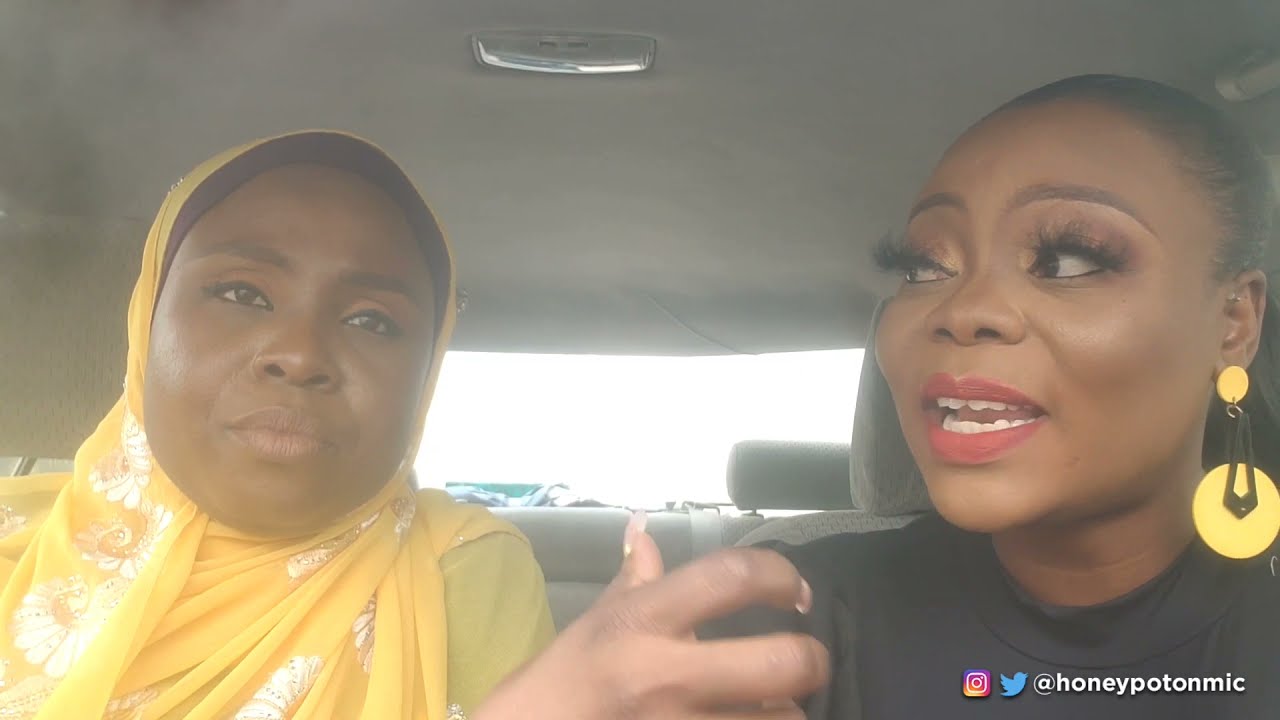The image captures two African-American women with darker skin complexion sitting in the front seats of a car during daytime, as natural light streams in from the rear windshield. The woman on the right, who is speaking, is dressed in a black shirt, has her hair slicked back, and wears striking goldish-yellow and black earrings along with long eyelashes and red lipstick. The other woman, who is listening, dons a yellow head wrap adorned with white flowers, complementing her green shirt, adding to the black and yellow color theme seen in this image. The interior features of the car, including the roof and upper dome light, are visible. Additionally, the bottom right-hand corner of the image shows the Instagram and Twitter logos, along with the username "@honeypotonmic," indicating that the image is a screenshot from an Instagram video.